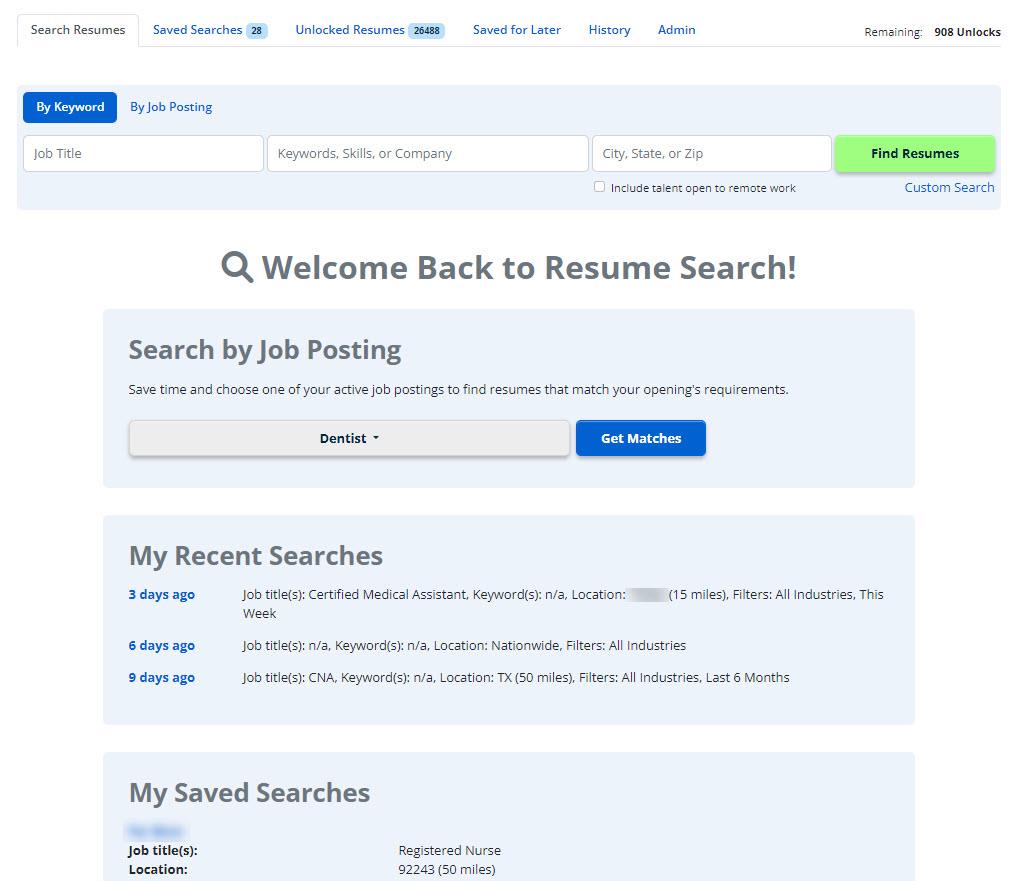The image displays a webpage interface for a resume search platform. At the top of the page, there are several tabs: "Search Resumes", "Saved Searches", "Unlocked Resumes", "Saved for Later", "History", and "Admin". Located in the upper right corner, the interface indicates "Remaining: 908 unlocks". Below these tabs lies a search section, where users can input keywords. To the right of this search bar is a prominent green "Find Resumes" button. Beneath this section, a welcome message reads, "Welcome back to Resume Search". Additionally, users are offered the option to search by job posting, with "Dentist" selected in the drop-down menu. There is also a "Get Matches" button for retrieving relevant resumes. The page further includes sections labeled "My Recent Searches" and "My Saved Searches" towards the bottom.